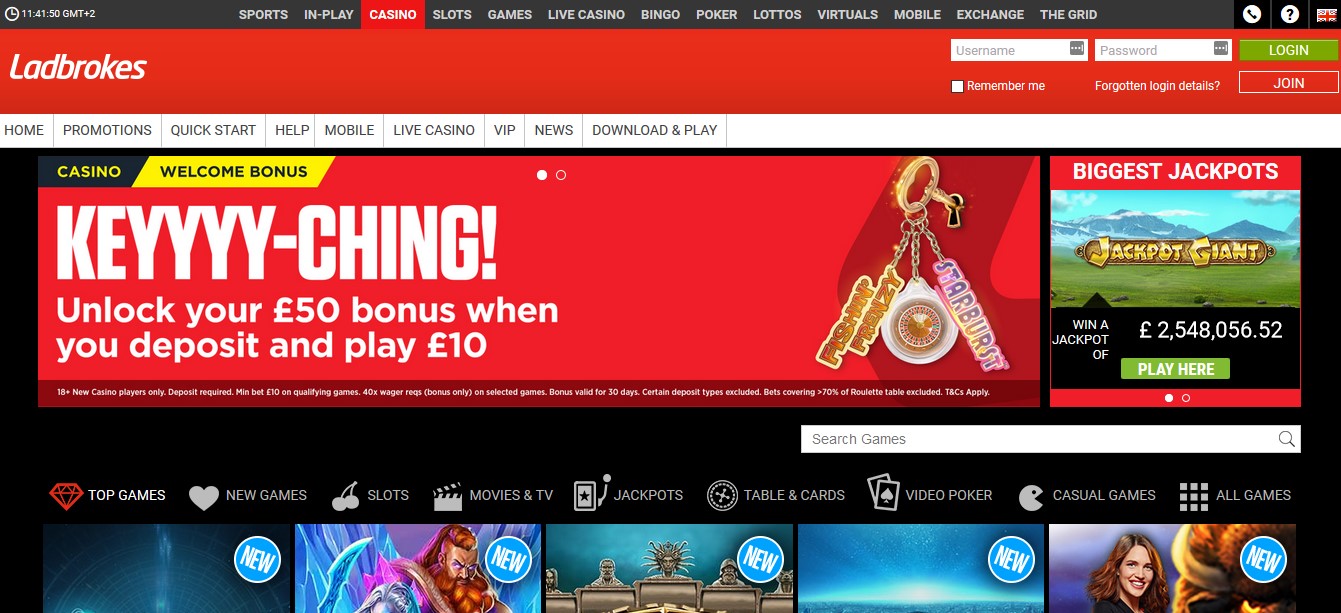The website appears to be for an online betting and gaming platform, likely Ladbrokes. 

At the top, there's a thin black banner featuring a round white circle displaying a clock with hands pointing to three o'clock. Next to the clock, text indicates the current time as "11:41:50 GMT+2." 

Directly below, a horizontal menu offers various options including "Sports," "In Play," "Casino," "Slots," "Games," "Live Casino," "Bingo," "Poker," "Lottos," "Virtuals," "Mobile Exchange," and "The Grid." Icons for customer support, such as a telephone and question mark, are displayed within circles.

The "Casino" menu item is highlighted with a red background and white text. Beneath the menu bar, the Ladbrokes logo is prominently displayed in bold, with links for "Username," "Password," "Login," "Join," "Remember Me," and "Forgotten Login Details" on the right.

The next section has another horizontal menu displaying options like "Home," "Promotions," "Quick Start," "Help," "Mobile," "Live Casino," "VIP," "News," and "Download and Play" in white text.

The main content area is headed with the word "Casino" in bright yellow text against a black background. Below this, a promotional banner offers a welcome bonus with black text on a bright yellow background. Another promotional graphic on a red background with white text reads "KEY-CHING: Unlock your £50 bonus when you deposit and play £10." Various other graphics and promotional images are also scattered throughout the page.